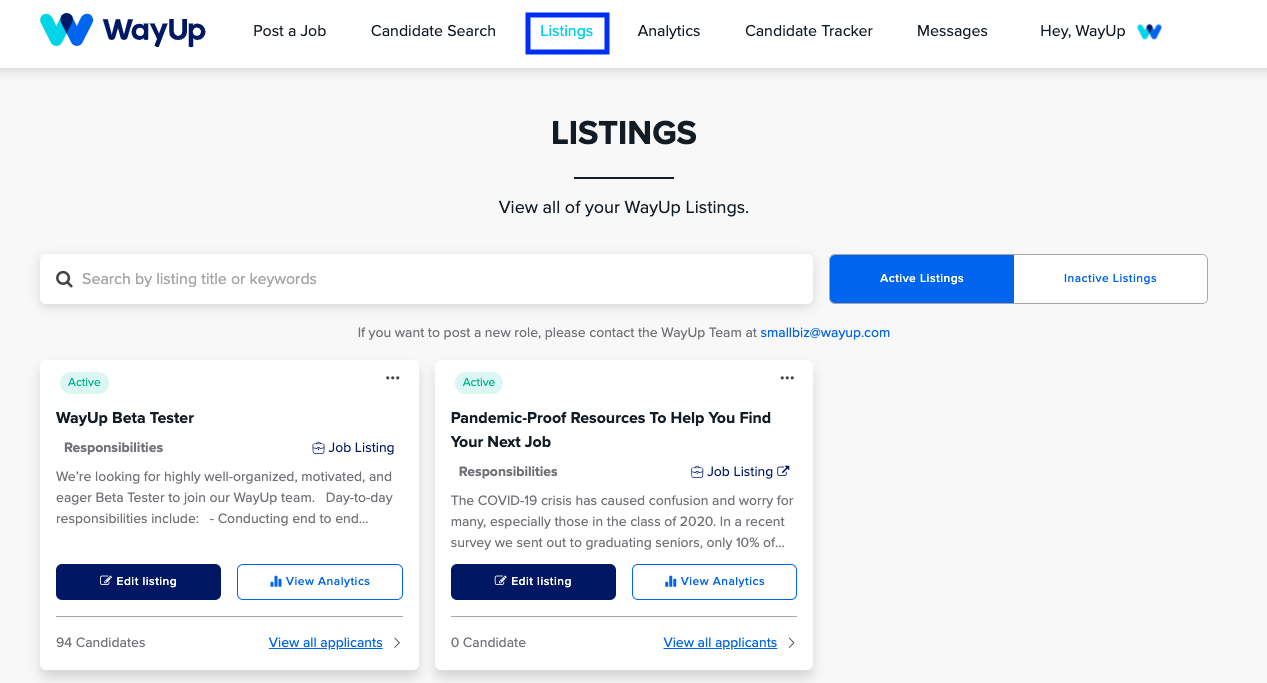**Caption:**

The homepage of the WayUp Listings platform features a clean, off-white background and a well-organized layout. At the top, there is a full-width rectangular white banner. In the far left corner of this banner is the WayUp emblem, which is a multi-shaded blue 'W'. Next to it, bold navy blue text spells out "WayUp," followed by smaller black text options including "Post a Job," "Candidate Search," a blue-outlined rectangle with blue text that says "Listings," "Analytics," "Candidate Tracker," "Messages," and finally, "Hey WayUp," accompanied again by the smaller WayUp emblem.

Centered below this banner, bold black text announces "Listings," with a thin line running horizontally beneath it. Below this line, in small black text, it reads, "View all of your WayUp listings."

Underneath this section is a prominent long white search bar that spans from the left to the middle of the screen. Inside this bar, starting from the left, is a black magnifying glass icon followed by placeholder text that reads, "Search by listing title or keywords." To the right of this search bar are two clickable rectangular options: a blue rectangle with white text saying "Active Listings," and a white rectangle with blue text saying "Inactive Listings."

Further down, a note provides helpful information: "If you want to post a new role, please contact the WayUp team at smallbiz@wayup.com."

The main content area displays two active listings side by side. The first square lists the role "WayUp Beta Tester" with its associated responsibilities. At the bottom of this square are two buttons: one for "Edit Listing" and another for "View Analytics." The second square features the listing "Pandemic-Proof Resources to Help You Find Your Next Job," with the same two buttons at the bottom for "Edit Listing" and "View Analytics."

This detailed layout ensures users can easily navigate through the platform to manage and view their job listings effectively.